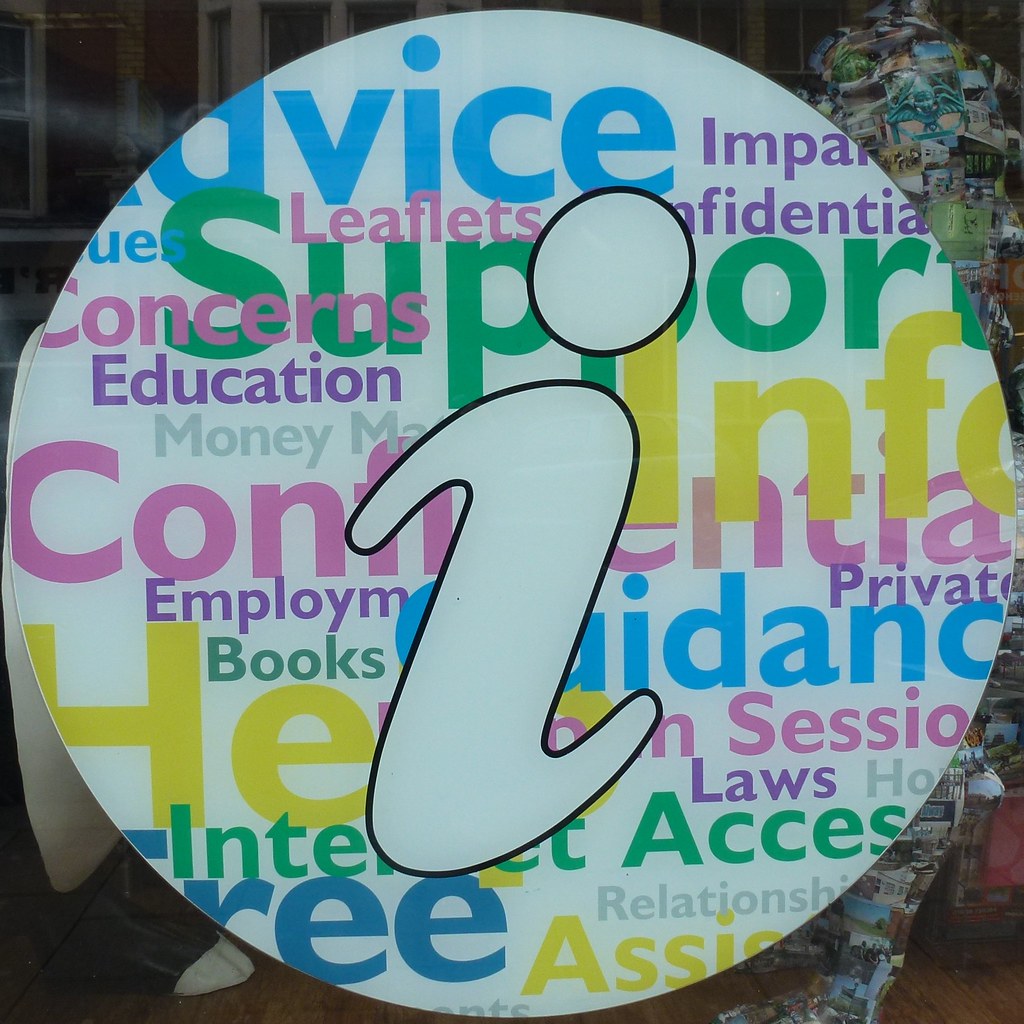This photograph, taken through a glass window with reflections hinting at an outline of a car and neighboring buildings, captures a prominent round white cutout, likely made of cardboard. The cutout is densely covered with various vibrant words in pastel colors—blue, pink, purple, yellow, and green—reading "vice," "leaflets," "support," "competitive," "books," "employees," "laws," "access," "free," "education," "concerns," "employment," "private," "confidential," "internet," "guidance," and "relationships." Dominating the center of this cutout is a large lowercase "i," white with a black outline. Behind this intricate display stands a mannequin, strikingly covered head-to-toe in hundreds of photographs, adding an intriguing visual texture. The window's reflections obscure much of the interior details, though glimpses of an adjoining building's windows are visible in the top left corner.